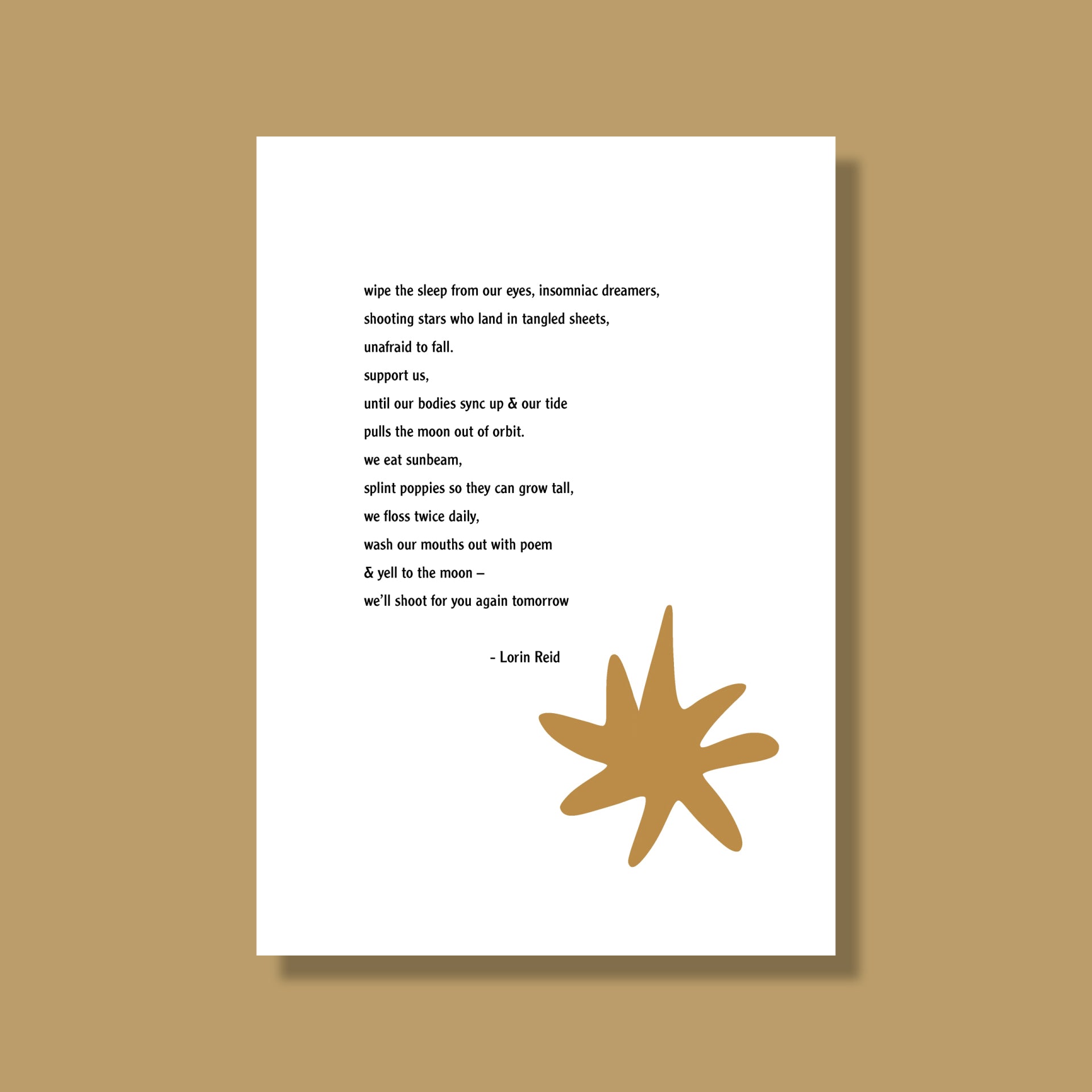The image depicts a digital design resembling a Microsoft PowerPoint presentation, featuring a white plaque over a camel-colored background. Centered on the white plaque is a poem in bold black text by Lauren Reed. The poem poetically speaks to "insomniac dreamers," urging them to "wipe the sleep from our eyes," and describing "shooting stars who land in tangled sheets, unafraid to fall." It continues with vivid imagery: "support us until our bodies sink up and our tide pulls the moon out of orbit," and "we eat sunbeam, splint poppies so they can grow tall." It also mentions daily rituals: "we floss twice daily, wash our mouths out with poem and yell to the moon, we'll shoot for you again tomorrow." Below the poem, the author's name is printed. The plaque features a camel-colored design that appears to be a star or leaf pattern, blending harmoniously with the camel-colored background.